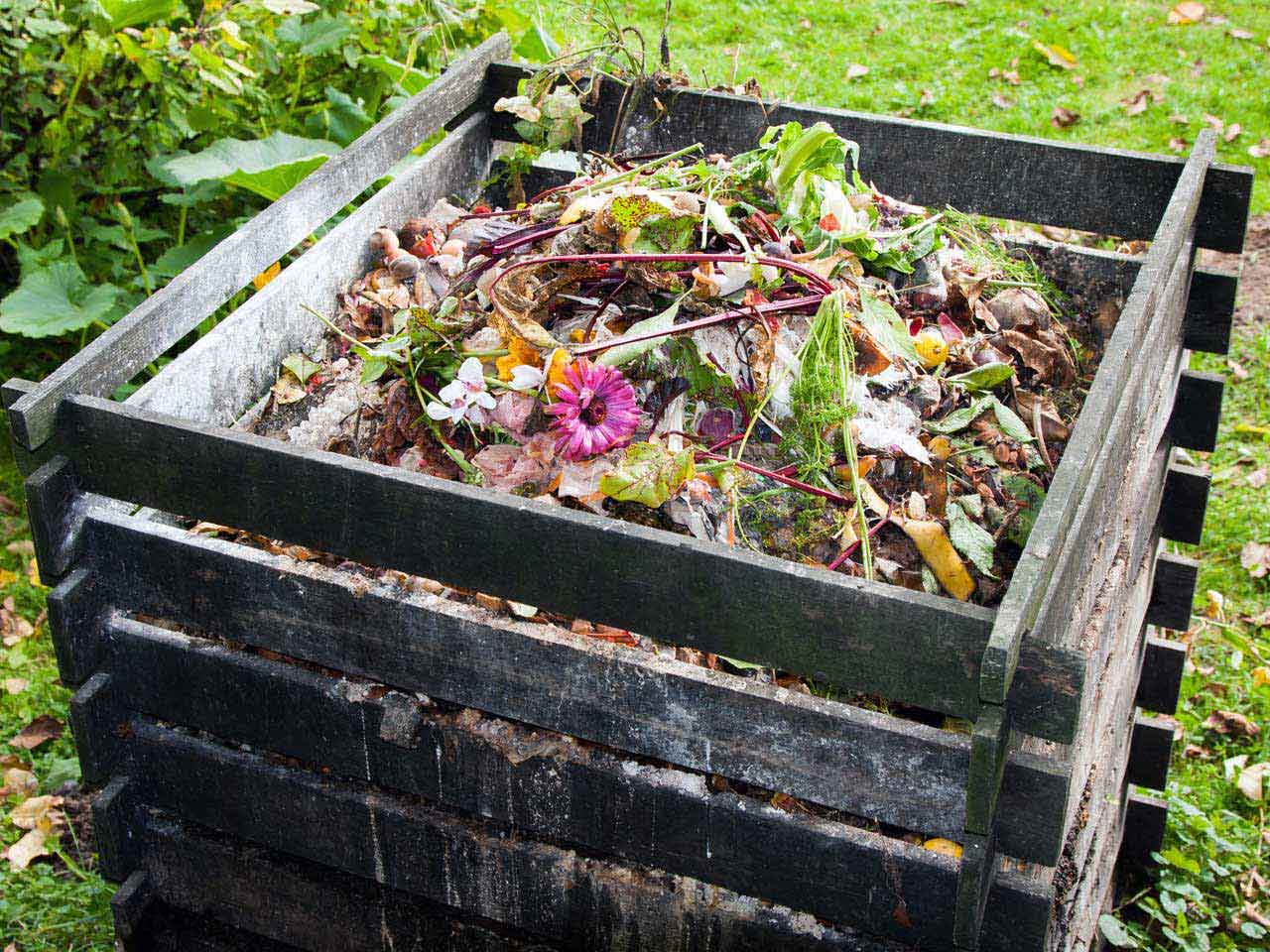This detailed, rustic close-up captures a beautiful compost pile contained within a weathered, wooden crate, made of gray, discolored slats with wide openings. The crate rests on a grassy yard, surrounded by several large leafy plants, possibly from squash or watermelon vines. The compost heap itself is a vibrant mosaic of organic matter, featuring a mix of vividly colored green and dried leaves, carrot and beet greens, and bright flower blossoms such as mums and forget-me-nots. Intriguingly, there are also strips of fruit and rhubarb among the composted waste, spilling slightly through the gaps in the crate. The surrounding area frames the compost pile with brown leaves scattered on the grass, creating a picturesque garden scene.